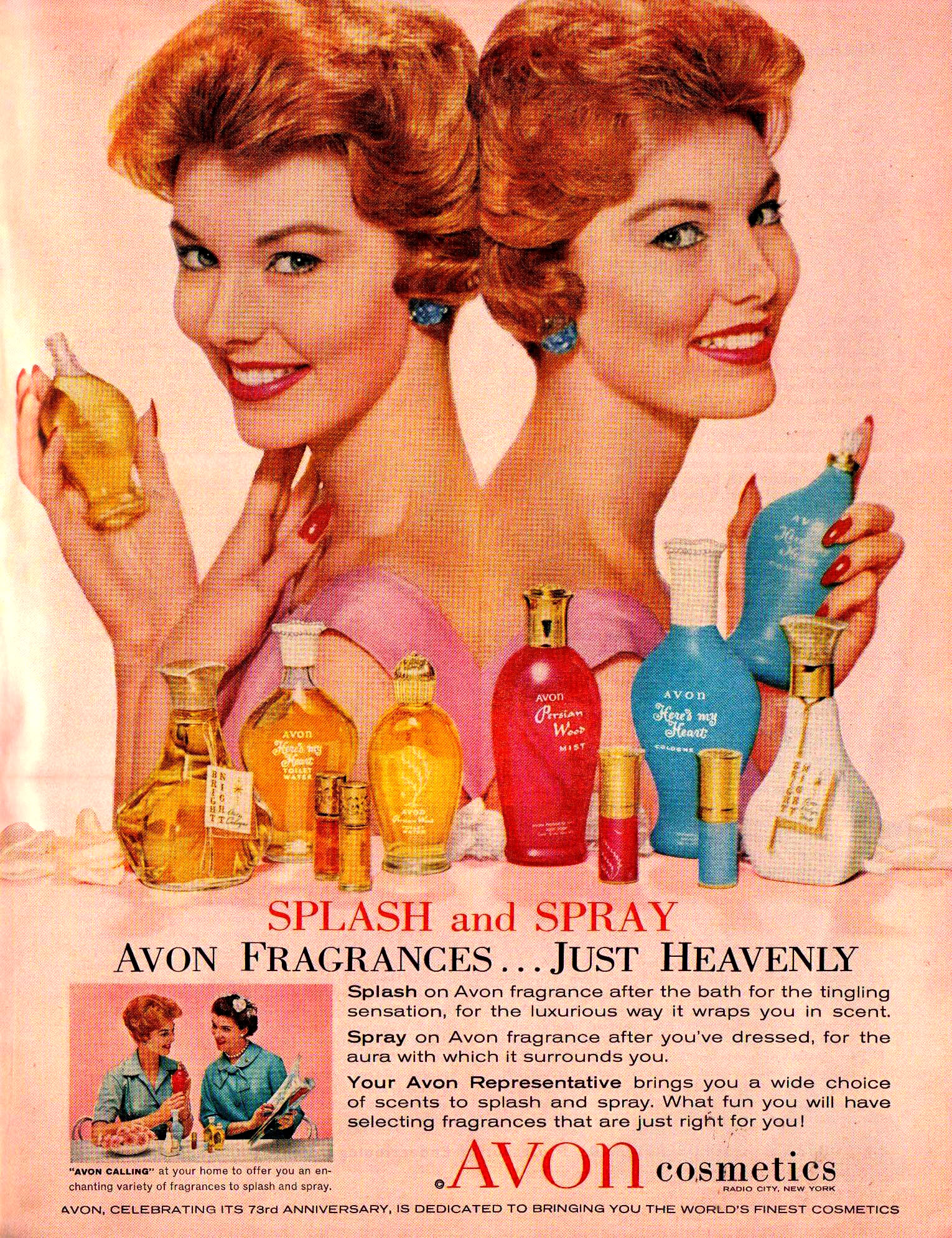This vintage Avon advertisement, possibly from the late 1930s or 1940s, prominently features a red-haired woman standing back-to-back with her mirror image, creating the illusion of twin figures. Both identical figures don a pink dress, accessorized with blue earrings, red nail polish, and vibrant red lipstick. The woman’s short, curly hair is meticulously styled, giving her a classic, timeless appearance. In her right hand, the figure on the left holds a yellow perfume bottle, while her counterpart on the right grasps a blue bottle.

The header of the ad reads “Splash and Spray, Avon Fragrances… Just Heavenly.” Beneath this inviting title, a descriptive paragraph encourages the use of Avon fragrances both after the bath for a lasting luxurious scent and after dressing for an encompassing aura. The ad enthusiastically suggests that selecting and using these fragrances will be an enjoyable and personal experience. 

Towards the bottom left of the page, there's a smaller inset image depicting two women testing out the perfumes, engaging in a friendly evaluation of the scents. Below this smaller image, the wording reads “Avon Cosmetics,” followed by a celebratory note indicating Avon’s 73rd anniversary, emphasizing the brand’s commitment to providing the world's finest cosmetics.